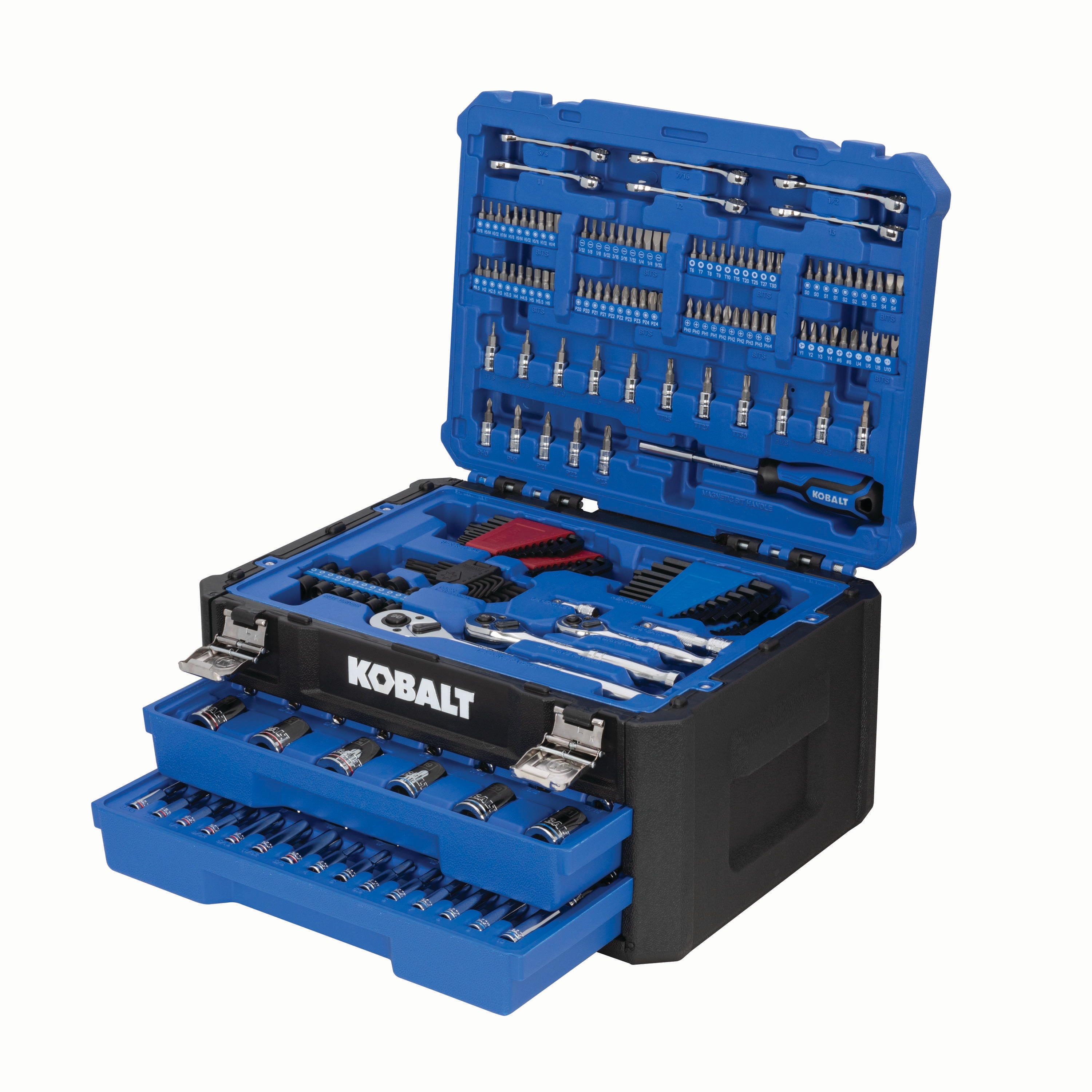The image features a meticulously organized toolbox with a distinct color scheme of black and blue. The sides of the toolbox are black, while the front is accentuated with a black stripe, followed by a blue base. The toolbox includes several compartments which can be opened, resembling shelves or drawers. 

In the top drawer, there are six circular items neatly arranged. The lower drawer contains numerous slimmer items compared to those in the top drawer. On the very top layer of the toolbox, the blue background contrasts with an assortment of tools, including pliers, red, silver, and black items, and various implements. 

Additionally, the inside of the lid also has a blue backdrop, housing several more tools against it. Notably, a blue-handled screwdriver is among the items inside the toolbox, contributing to the organized yet varied collection of tools.